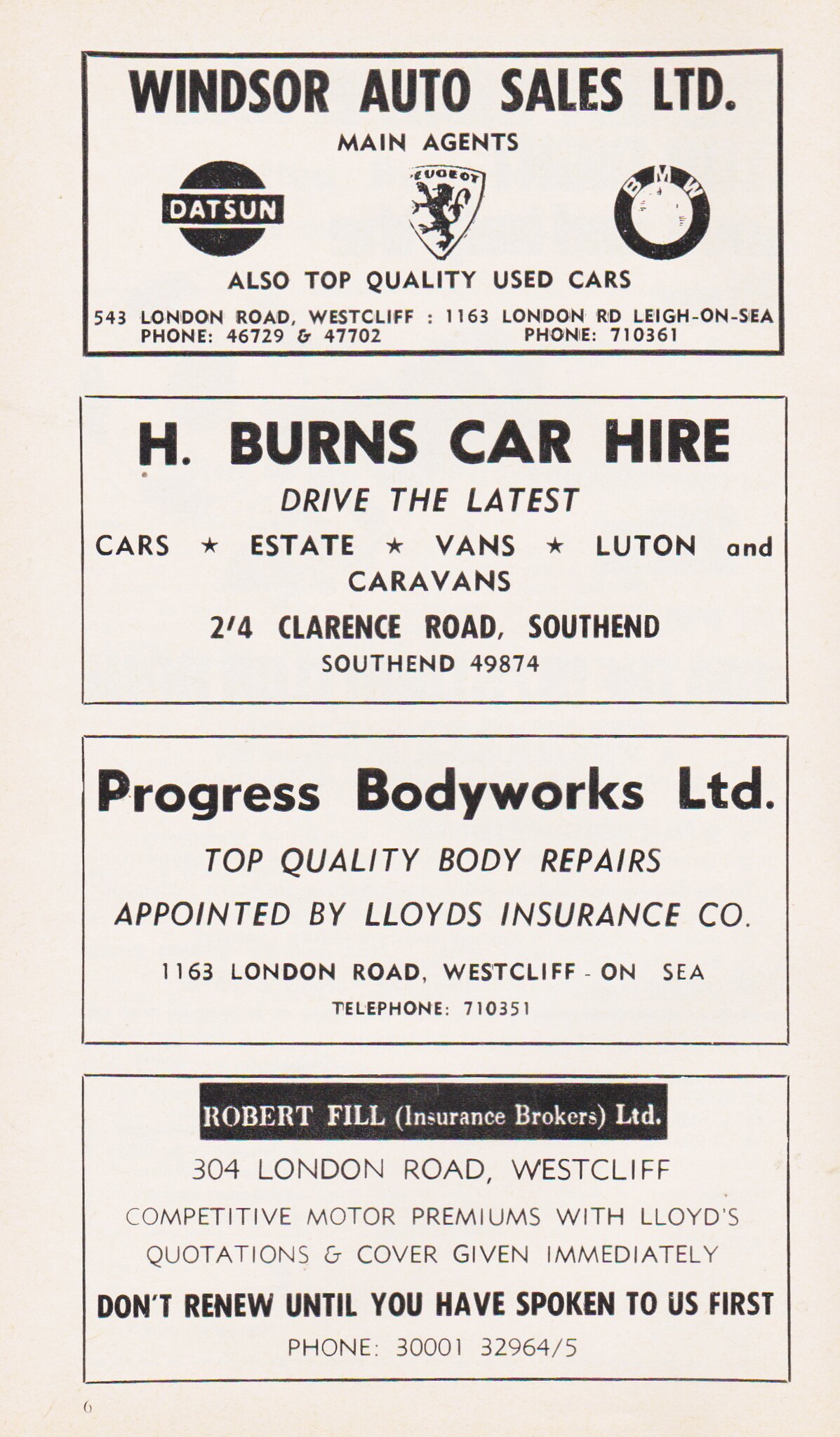This image, reminiscent of a newspaper advertisement page, showcases four neatly separated ads against a cream background, each within its own rectangular panel. The top panel belongs to Windsor Auto Sales LTD, highlighting their status as main agents for Datsun, BMW, and Peugeot. It promotes "top quality used cars" and provides contact details. The second panel is for H Burns Car Hire, offering a range of vehicles including cars, estates, vans, Luton models, and caravans, along with their address. The third advertisement, from Progress Body Works LTD, emphasizes "top quality body repairs" and mentions their appointment by Lloyd's Insurance Company, including an address and a telephone number. The bottom panel features Robert Phil Insurance Brokers LTD, prominently located at 304 London Road, Westcliff, boasting "competitive motor premiums with Lloyd's quotations and cover given immediately." It advises prospective clients to consult them before renewing any insurance, with contact details provided beneath.